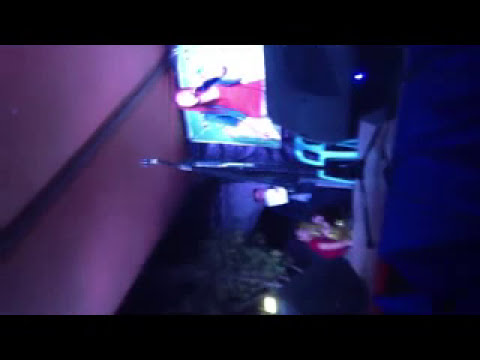This image appears to be a very blurry, low-quality, pixelated, and out-of-focus photograph, requiring a 90-degree rotation for correct orientation. The scene features a woman who appears to be Caucasian with long hair down to her shoulders. She is wearing a red shirt and possibly a blue sweater. She is holding what seems to be a microphone, standing on what seems to be a stage with large speakers and a microphone stand in front of her. The setting suggests she might be giving a speech, such as a wedding toast, or performing a comedy act. There are two other people in the image: one crouched down wearing red and another person's face visible behind. Further details include a possible TV or monitor, a table with an object, a ceiling with purple coloration, and light obscuring parts of the scene. The overall setting could be the inside of a club or another type of indoor venue. Colors observed in the image include tan, purple, black, gray, red, green, yellow, and white. The majority of significant elements are clustered towards the center of the photo, and though there is no text, the scene suggests a gathering or public event indoors.